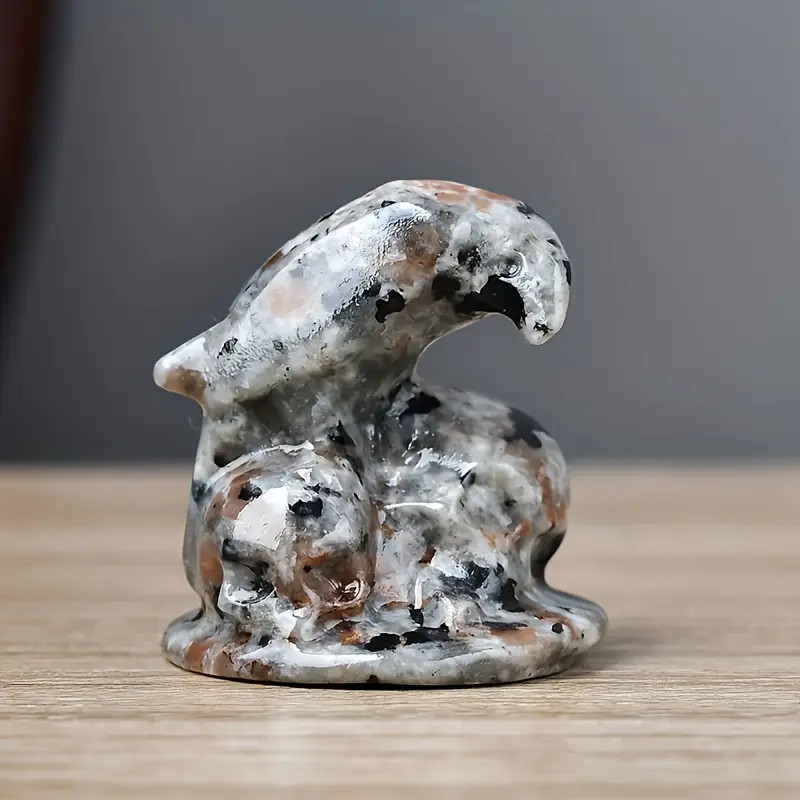The image is a close-up photo of a small, intricately worked sculpture, likely composed of marble or a similar crystalline material. Held within the palm of a hand, the sculpture exhibits a blend of brown, grey, black, and nearly transparent hues, enhancing its abstract yet evocative nature. It predominantly features what appears to be a bird, possibly a parrot, characterized by its curved beak directed towards the viewer. The bird is perched atop a formation resembling a stone, which bears an impression that could be interpreted as a skull on the left side. Interestingly, the base of the sculpture also hints at the form of a dog or possibly even a dolphin, adding to the ambiguity and complexity of the piece. This fusion of motifs encourages contemplation of themes such as eternity and mortality. The sculpture rests on a light brown wooden table, with a plain gray wall serving as the backdrop, characteristic of a gallery setting which isolates the art, inviting focused attention on its details and form.